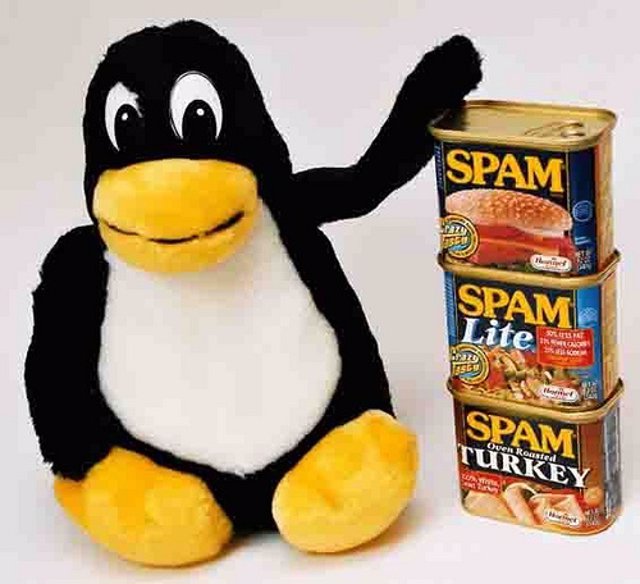The photograph features a stuffed penguin sitting on a white surface against a white background. The penguin, primarily black, boasts a white chest and belly, yellow beak, and matching yellow feet. Its big black eyes gaze towards the right side of the image. The penguin's left wing rests on a stack of three cans of Spam, identified from bottom to top as Spam Oven Roasted Turkey, Spam Light, and the original Spam, each with a gold top and blue front label. The penguin appears content next to the neatly stacked cans, vividly detailed in the image.